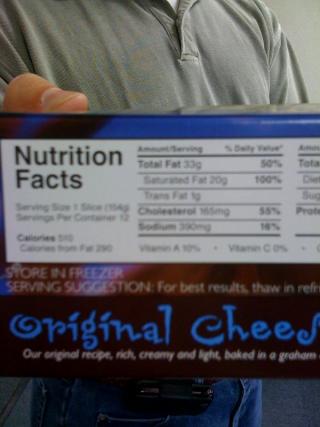A man, wearing a gray polo shirt and blue jeans, is depicted holding a box with his right hand, but only his thumb is visible in the top left corner of the image. The man himself is seen only up to his neck, as his head is cut off from the frame. The box he's holding features a nutrition facts label on the back, printed in black ink on a white surface. Below the nutrition label, partially obscured text reads "original cheese," with the final "e" missing. Additional text mentions "original recipe, rich, creamy, and light," but is cut off further along, with "baked in a gram" similarly truncated. The phrase "original cheese" is styled in a fancy blue script against a black background, while the remaining text is in white. The box's upper edge has a blue label accented with dark brown, resembling a flowing, melting chocolate design. The incomplete label further directs to "store in refrigerator" and a serving suggestion that is also partially cut off.